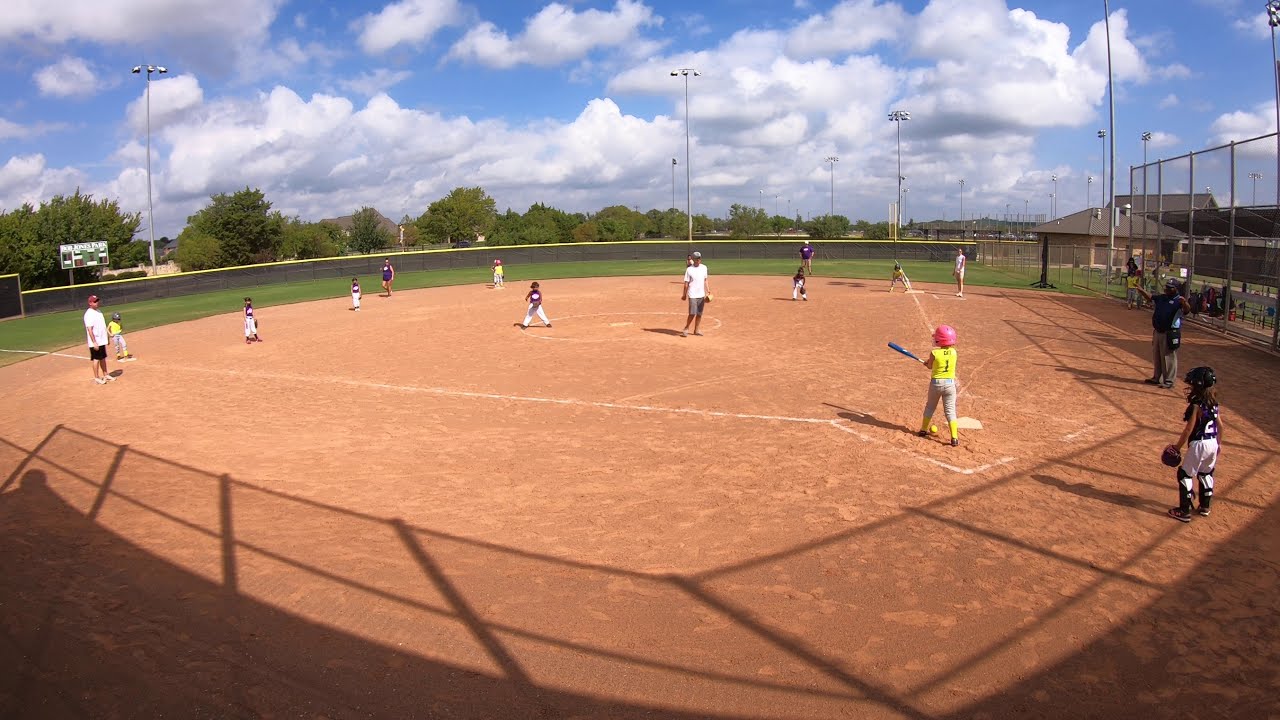Under a vibrant blue sky decorated with fluffy clouds, a lively little league baseball game unfolds on a well-maintained field. At home plate, a small child wearing a red helmet and a yellow shirt with the number one stands mid-swing, holding a blue or purple bat. An adult, likely a coach, stands on the mound pitching, while another adult, possibly the coach or umpire, observes from behind. The field is dotted with young players in purple shirts and white pants, spreading out over the verdant green grass.

To the left, at third base, another child stands poised, wearing a little red baseball hat, a long white t-shirt, and black pants, possibly a coach. Behind this scene, a distant scoreboard hovers over the field, difficult to read but clearly indicating the game is still in progress. In addition, light posts and other fields in the background suggest this is part of a larger athletic complex.

Despite their young age, the players seem deeply engaged in the game, while adults positioned near first base, third base, and scattered around watch attentively. The catcher is seen standing behind the batter, appearing ready to catch a pitch or observe the ball's trajectory just after a potential hit. Surrounding the field, one can spot trees, houses, and shrubbery, adding to the picturesque setting of this sunny, joyful afternoon of America's pastime.